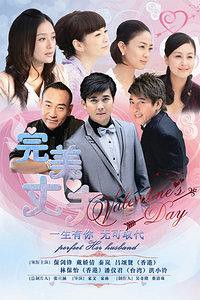This is a poster for an Asian film or TV show, possibly Thai, centered around Valentine's Day. The design features a striking light blue background with light pink in the center, accented by swirls of red. Dominating the top half of the poster are four women seen from the chest up, all gazing off to the side. Two of these women have medium-length hair, while the other two have shorter styles. Below them are three men, all in suits, looking directly at the camera. They all have short hair, with one appearing older than the other two. Across the bottom third of the image, there's a lot of text resembling movie credits. The most prominent text reads "Valentine's Day" in dark red cursive, positioned in front of the two rightmost men. Additional smaller text is present but too hard to read. The overall layout and composition suggest a romantic theme set against a visually engaging backdrop.